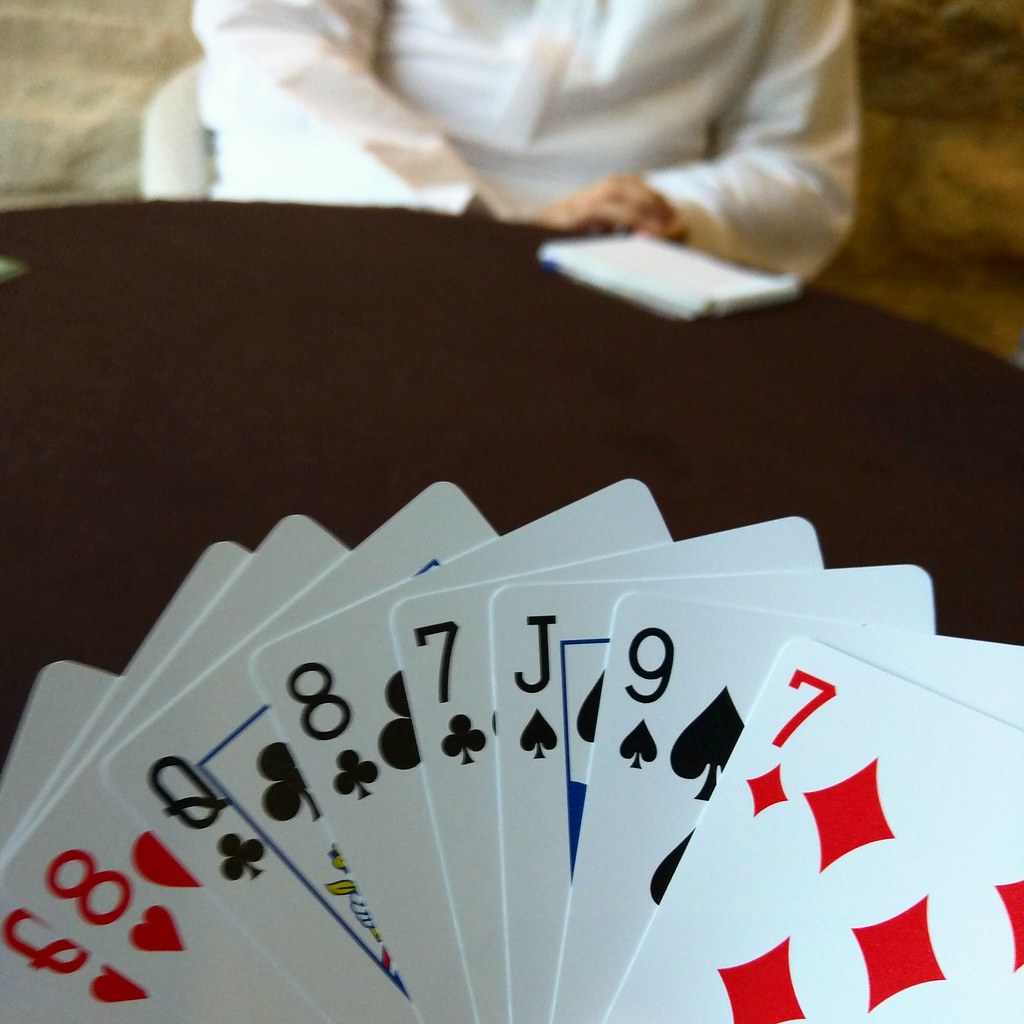The image captures a close-up view of a hand of playing cards from the perspective of the player. In the player's hand, from right to left, the cards are the Queen of Hearts, Eight of Hearts, Queen of Clubs, Eight of Clubs, Seven of Clubs, Jack of Spades, Nine of Spades, and Seven of Diamonds. There is a partially obscured card behind the Queen of Hearts. The scene is set against a round brown table. Across the table, another person is seated on a white chair, wearing a long-sleeved white shirt. This person has no cards in hand but has a white notepad and possibly a pen in front of them. The background features abstract swirls of brown, khaki green, and tan colors.